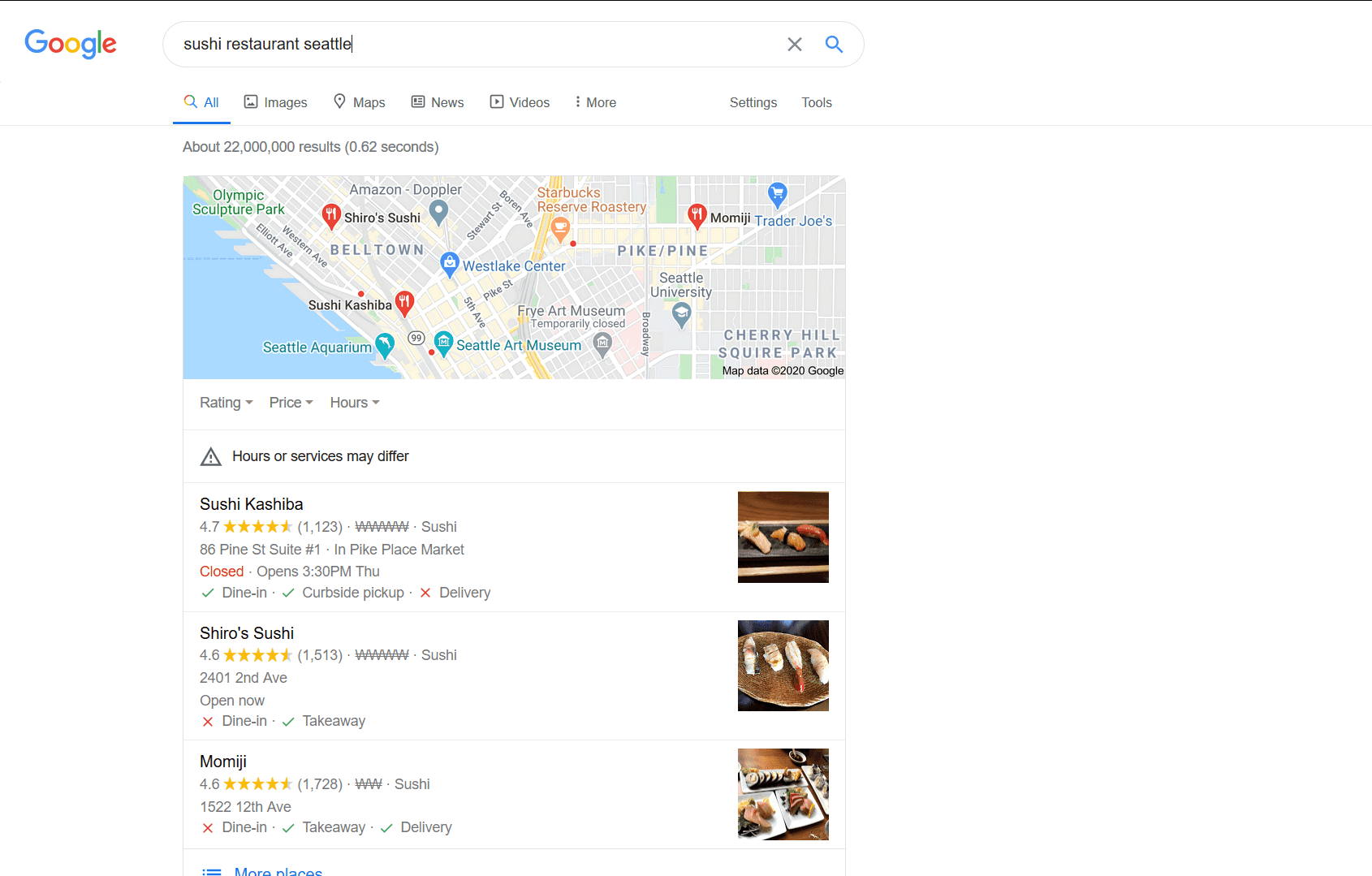The image showcases a Google search results page for "sushi restaurants in Seattle." At the top, the interface features various tabs such as "All," "Images," "Maps," "News," "Videos," and "More." Below, it displays the total number of search results and presents a map indicating different sushi restaurant locations.

The search results provide detailed information for three restaurants: 

1. **Sushi Kashiba** - Rated 4.7 stars.
2. **Shiro's Sushi** - Rated 4.5 stars.
3. **Momiji Sushi** - Rated 4.5 stars.

Adjacent to the listings, each restaurant's entry is accompanied by an image showcasing their sushi and the interior of the restaurant. Additionally, there's a note indicating that the business hours and services may vary, and a six-hour time frame is mentioned, although it's unclear what it specifically refers to.